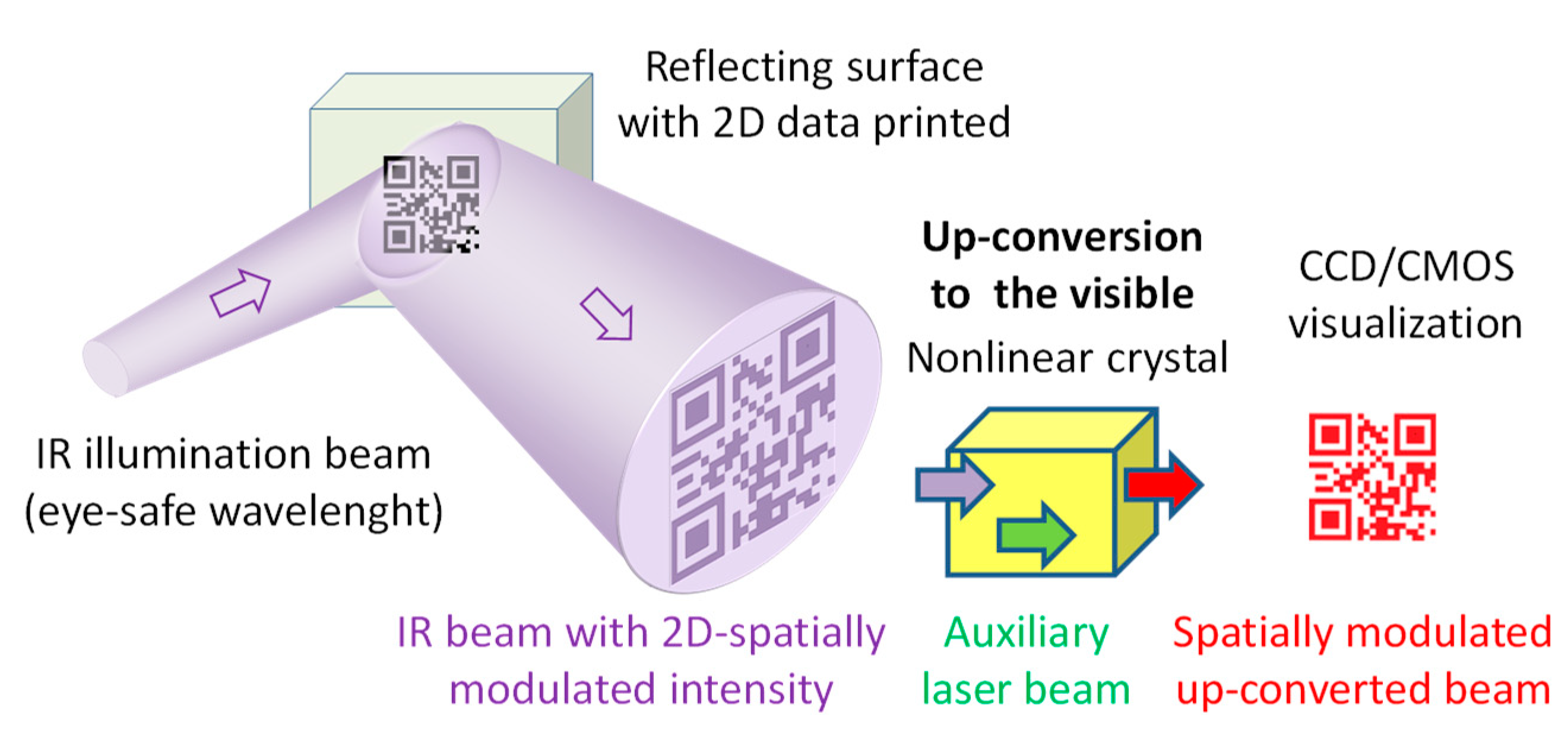The image showcases an informative chart illustrating the process of light beam modulation and visualization. It includes extensive text and three key pictures. The first picture is a cone-shaped object covered with several QR codes, depicted in purple. The second picture is a yellow box featuring three arrows in purple, green, and red, indicating the direction of light travel. The third picture is a red QR code. The chart details steps involving an IR illumination beam and a reflecting surface with 2D data. The text includes terms like "IR illumination beam," "2D spatially modulated intensity," "up conversion to the visible," "auxiliary laser beam," and "spatially modulated upconverted beam." It also references "CCD CMOS visualization" for visual representation. The diagram explains the modulation of IR beams to visible light using QR codes and makes use of various light beams and spatial modulations, providing a comprehensive overview of the process.